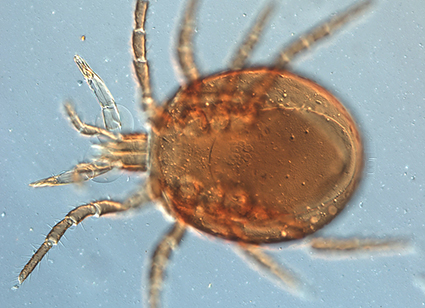The image depicts a brown, microscopic insect with a circular body, observed under a microscope. It is immersed in a liquid, indicated by the presence of tiny droplets and bubbles scattered throughout the frame. The insect, which could be a water bug or a tick, features eight legs—four extending towards the top and four towards the bottom of the image. Its antennae, shorter than its legs, also point leftward. The background is a light bluish-gray hue, enhancing the appearance of small white specks and bubbles in the liquid. The insect's body appears somewhat translucent, particularly at the extremities, resembling a tiny beetle or spider, with detailed segmentation visible in its legs.